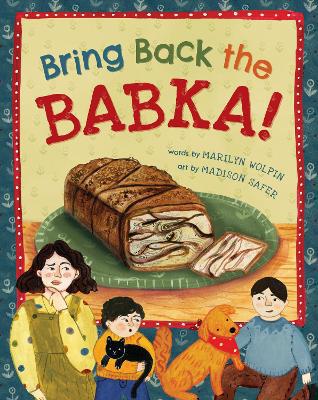The front cover of the children's book "Bring Back the Babka" features a playful and colorful design. The title, with each word in a different color—blue for 'Bring', green for 'Back', orange for 'The', and red for 'Babka'—stands out against a light yellowish background. Below the title, it states in blue lettering: "Words by Marilyn Wolpin, Art by Madison Safer." Central to the cover is an illustration of a loaf of babka, revealing its marbled interior of creams and browns, placed on a green plate set on a brown table. Surrounding this central image is a red band with white polka dots, and an outer border decorated with blue and white flowers. At the bottom of the cover, a woman with long brown hair and pale skin appears deep in thought, with her hand raised to her chin. To her right, a young boy in a yellow sweater holds a black cat, and next to him sits another boy, petting a brown dog with a red scarf. The expressions on all characters' faces convey curiosity and contemplation.